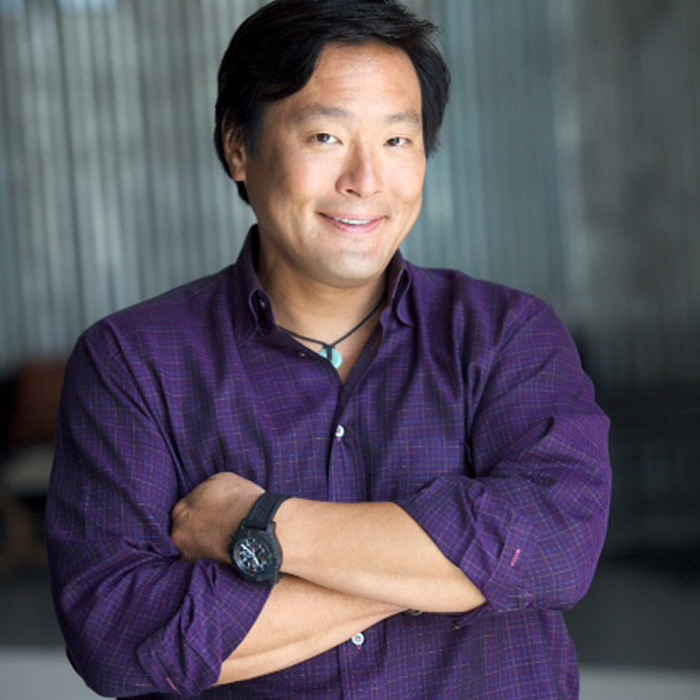In the center of the image, there's an Asian man with wavy, black, medium-length hair and dark brown eyes, looking directly at the camera with a warm smile. His eyebrows appear finely groomed. He is wearing a long-sleeved, button-up purple shirt with a striped and plaid pattern incorporating hues of blue and orange. The sleeves are rolled up to reveal a black watch with a black wristband on his left wrist. Around his neck, he dons a black necklace featuring a circular pendant, possibly jade. The man's arms are crossed over his chest. The background appears slightly blurry with sheer curtains in front of what looks like corrugated steel or metal walls, giving the impression of a professional photograph taken in an industrial setting.